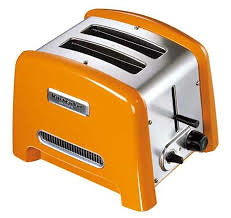The image depicts a stylish, vintage-inspired Japanese toaster. The toaster features a robust, square design with bright orange enamel on both of its sides, contrasting with a central body made of stainless steel. It is oriented diagonally in the image, with the controls facing the lower right corner. This two-slice toaster boasts a pair of wide slots on top, visible with a black interior.

On the front side of the toaster, which is fully orange, there's a distinctive silver label towards the bottom, inscribed with the brand name "MNIMAN" in black letters. Below this label, the orange panel includes a vent-like design with visible screws at the sides, adding to its retro aesthetic.

The right side of the toaster showcases a functional control area. It includes a black lever handle for lowering the bread into the slots and two black knobs: one for adjusting the browning intensity and another with an unclear purpose. The controls are set against a small oval panel beneath the lever. 

The clean white background highlights the toaster’s striking color and metallic details, making its modern-retro fusion style stand out vividly.